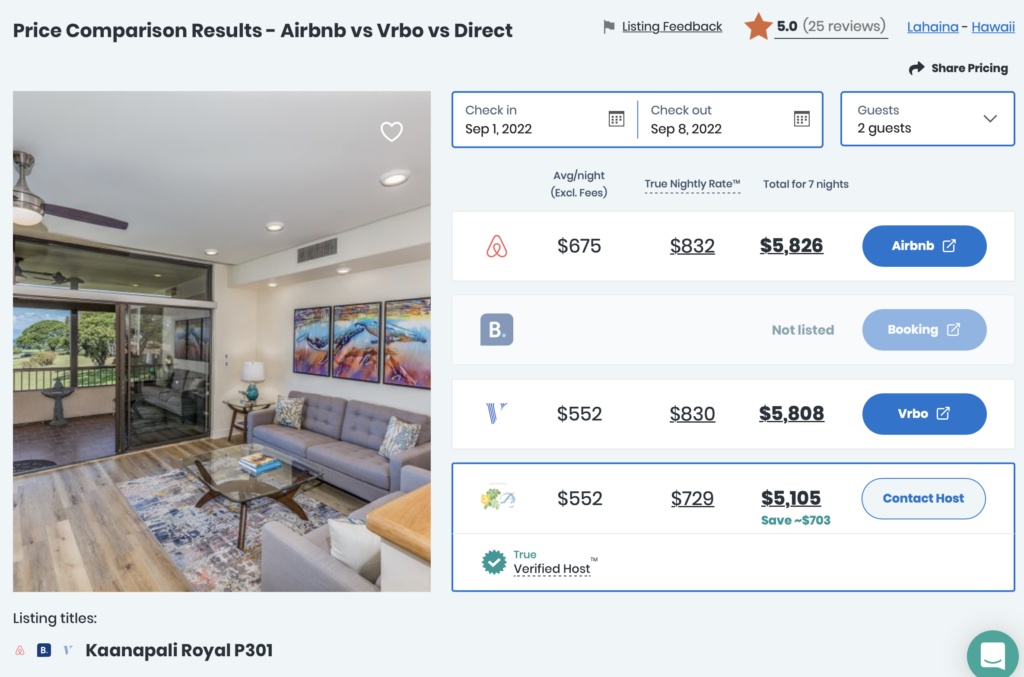The image depicts a detailed price comparison for short-term accommodations from three booking platforms: Airbnb, VRBO, and Direct. The backdrop is a light blue-gray color, setting a neutral tone for the comparison table displayed prominently in the center. At the top of the image, the title "Price Comparison Results Airbnb vs. VRBO vs. Direct" is written in black font, providing immediate context.

The comparison focuses on accommodations for a seven-day stay, from September 1st to September 8th, 2022, for two guests. The primary listing under scrutiny is "KANAPALI Royal P301." The nightly rates for this listing vary significantly: the most expensive option is $832 per night, while the cheapest is $729 per night. This variance affects the total cost for the week-long stay, which ranges from $5,105 to $5,826, excluding additional fees. The overall average price is somewhat lower but still substantial, indicating that this is a high-end accommodation choice.

The image's purpose is clearly to help the viewer make an informed decision by comparing costs across different booking platforms for a specific date range and accommodation type.